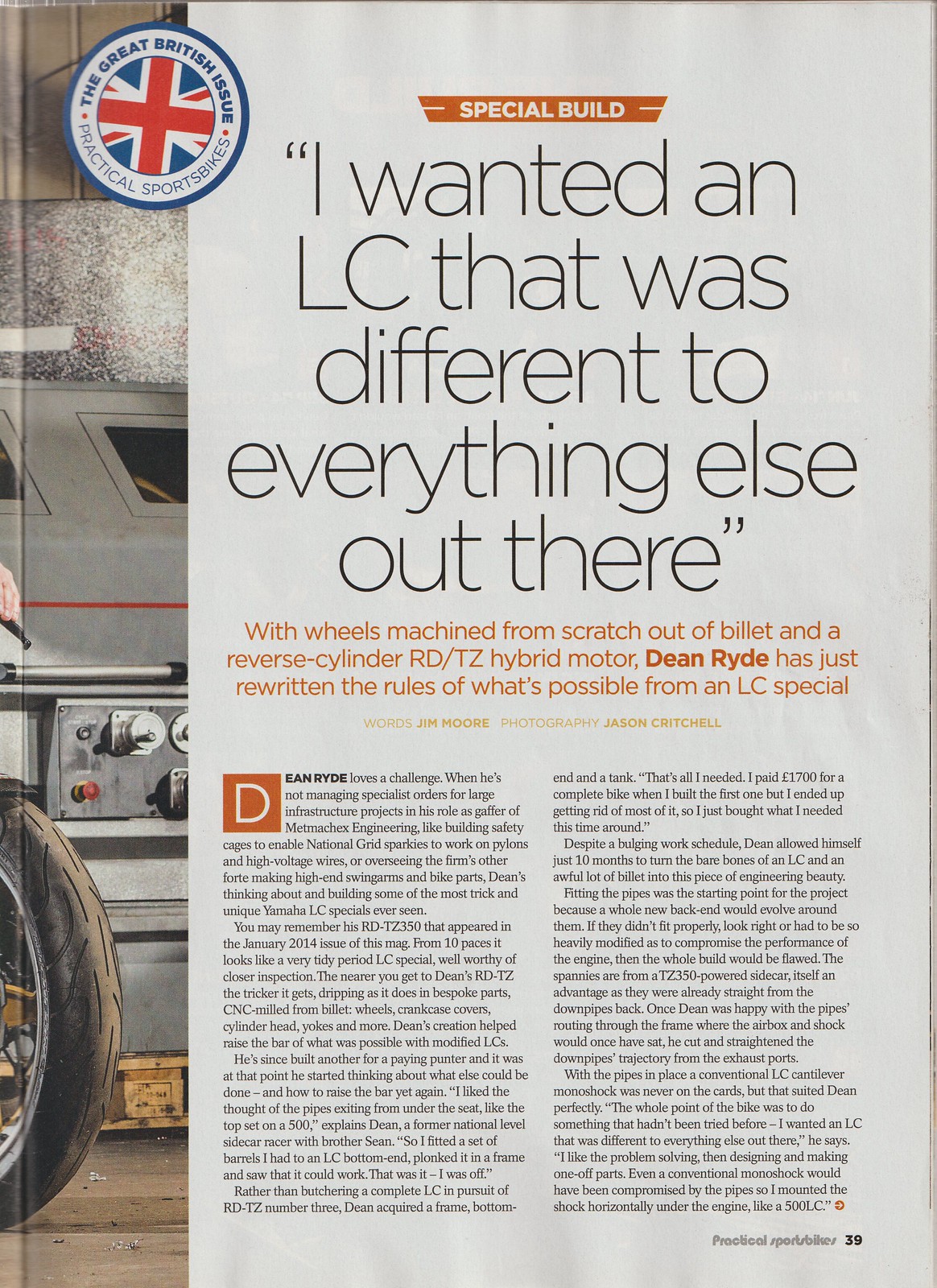The image shows a scan of a magazine page, specifically page 53, which appears folded under at the center. The background is predominantly white with features in black and red. At the top left of the page, there's a distinct circle with a Union Jack inside, encircled by a white band with the words "The Great British Issue" and a blue border around it. This badge denotes the magazine's special British-themed edition of "Practical Sports Bikes."

Dominating the top section of the right-side page is the title in bold black lettering, "I wanted an LC that was different to everything else out there," followed by a small red banner stating "Special Build" above it. Beneath the main title, in red text, it reads, "With wheels machined from scratch out of a billet and the reverse cylinder RD/TZ hybrid motor, Dean Ride has just rewritten the rules of what's possible from an LC Special." Dean Ride's name is in bolder red.

To the left of the text and partially visible due to the fold, there is a black tire and some metallic components, possibly motorcycle instrumentation. The body of the article is printed in two columns with very small text, making details hard to discern. The bottom right corner of the page features the number 53.